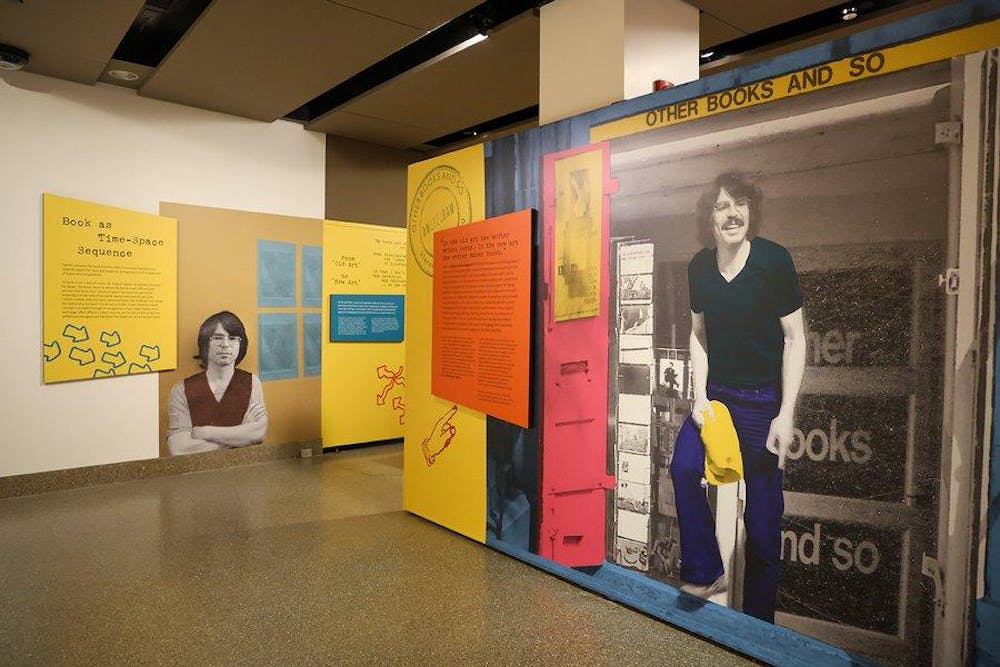In this detailed museum exhibit, we're looking at a vibrant room with white walls, black or brown speckled cement floors, and a dark ceiling. The exhibit, rich in color and design, features multiple large posters and panels primarily themed in yellow, blue, orange, and pink hues. Central to the exhibit are two main posters on opposing walls. 

On one wall, there's a yellow poster titled "Books as Time-Space Sequence," highlighting a young man with long shaggy hair, glasses, a black shirt, blue jeans, and a mustache. He is depicted in two black and white photographs; one where he stands carrying a yellow piece of cloth and another where he crosses his arms, wearing a brown vest over a dark green shirt.

Facing this, another large poster reads "Other Books and Sew." The intriguing artwork gives an illusion of a man stepping out of the flat poster. He is shown in blue pants, with his arms transforming from black and white to a 3D effect, as if reaching out of the exhibit. His vintage appearance, with long hair and a mustache, ties into early 80s aesthetics.

Additional design elements include doodles of arrows and pointing fingers on various panels, perhaps guiding viewers to important information, and smaller posters with details, though their text remains illegible due to the image's low resolution. The cohesive yet varied color palette and playful 3D illusions create a dynamic and engaging viewing experience.